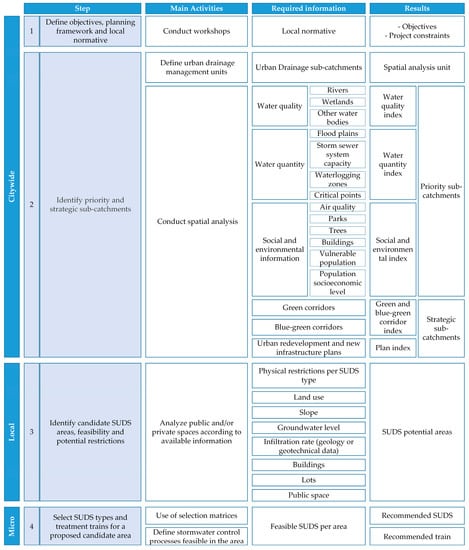The image is a detailed chart focused on city planning and water management processes, featuring a blue, white, and gray color scheme. The table is organized into columns with headers labeled "Steps," "Main Activities," "Required Information," and "Results." The rows are categorized under "Citywide," "Local," and "Metro." The tasks outlined in the chart include defining objectives, establishing a planning framework, and addressing local norms. Additionally, it highlights activities such as conducting workshops, managing drainage, and handling water analysis for rivers, wetlands, water quantity, and public spaces. This comprehensive document serves as a guideline for urban management, particularly focusing on drainage and water-related aspects across various administrative levels.